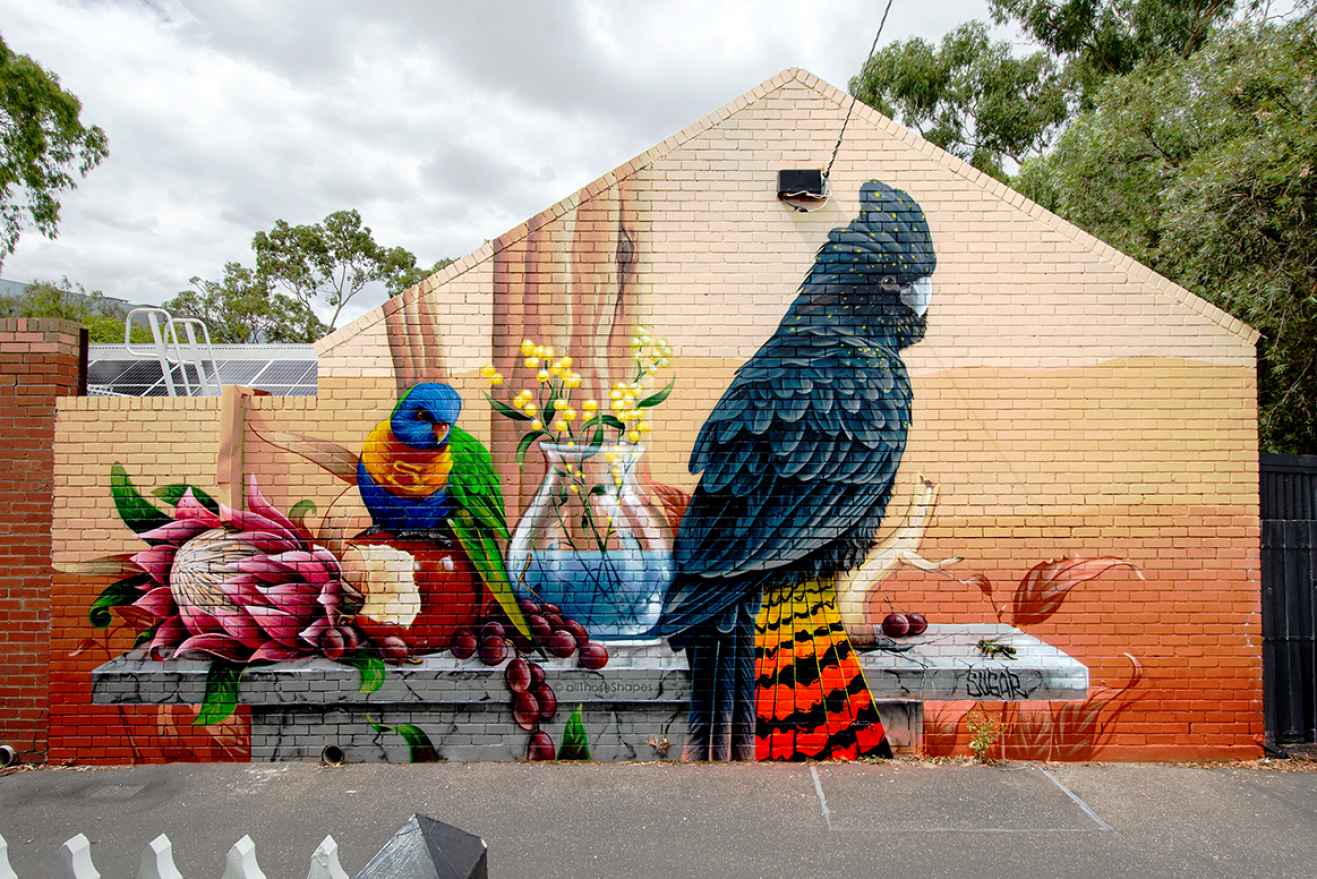This image features a detailed mural painted on the side of a brick building. The building has a flat surface on the right and culminates in a triangular roof. Grounded by an asphalt area, the vivid mural transforms the entire brick side into an artistic canvas depicting a still life on a stone table. 

Central to the mural are two birds. The bird on the right has striking blue feathers with a tail adorned in yellow and red with black stripes, resembling a cockatiel. To the left, perched on a partially eaten apple, is a parrot with a blue head, orange and blue body, and green wings and tail feathers. This parrot might have an orange chest according to another perspective. The still life composition also includes a large glass vase filled with blue liquid and white flowers, alongside an apple and a bunch of purple grapes.

The background of the mural mirrors the gradient of a sunset, transitioning from deep orange at the bottom through yellow and tan, culminating in a light beige or cream at the top. Surrounding the mural are depictions of trees and a richly colored sky. Adjacent to this mural, in the top right corner of the actual image, stands a real tree, further blending the painted scene with the natural environment. Additional background elements include clouds and possibly the edge of a ladder on the building's left side, hinting at a swimming pool nearby.

Overall, this mural intricately blurs the lines between art and reality, infusing a simple brick wall with vibrant life and color.